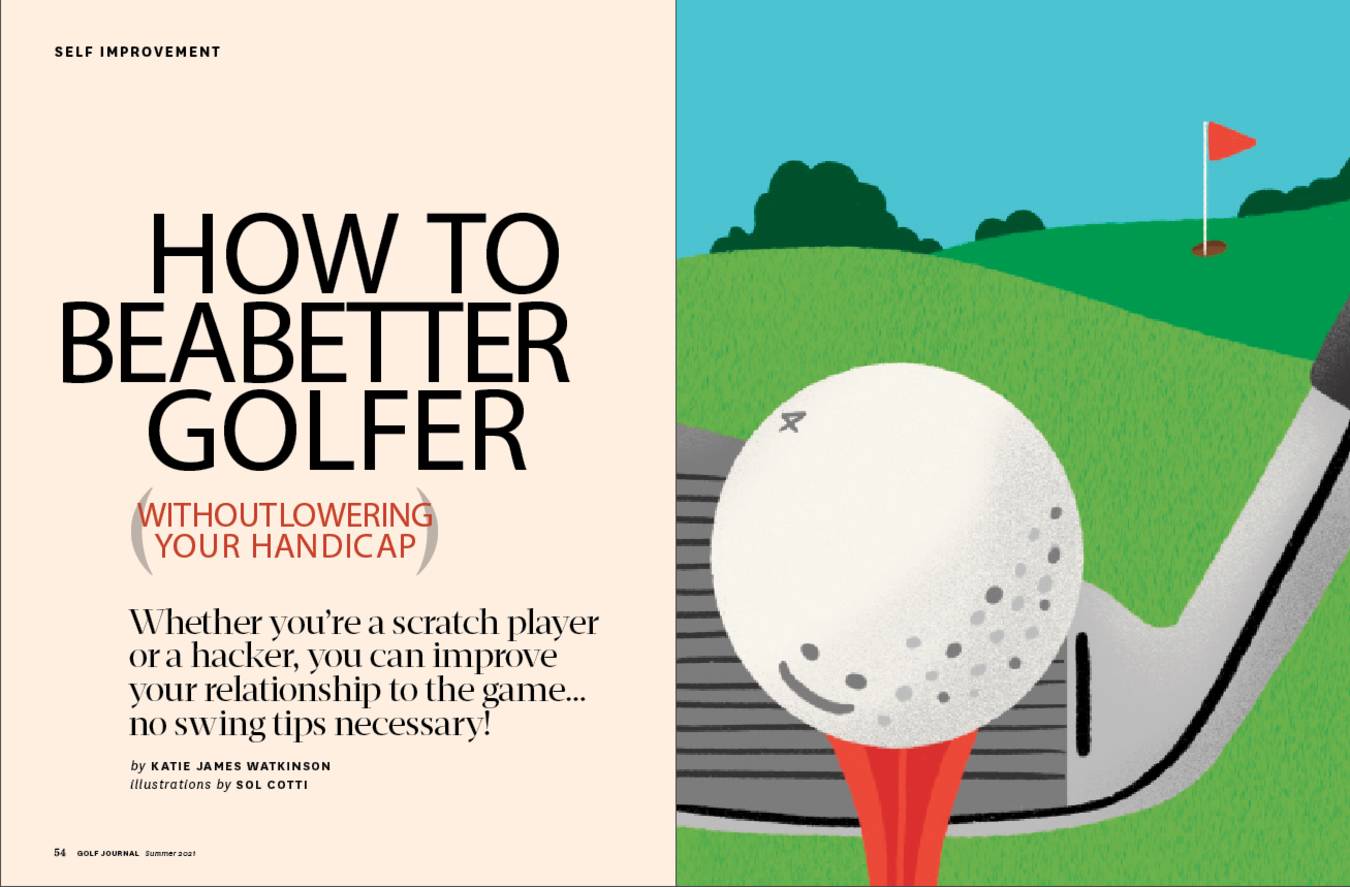This image is an interior page of a golf journal magazine, presenting a detailed and colorful advertisement. At the top left, the text reads "Self-Improvement," followed by the title "How to be a better golfer without lowering your handicap" on the left-hand side. It further explains, "Whether you're a scratch player or a hacker, you can improve your relationship to the game. No swing tips necessary." This article is authored by Katie James Watkinson with illustrations by Saul Cotty.

To the right of the text, there is a vibrant drawing depicting a golf course. A white golf ball with a smiley face, dotted with grey, sits atop an orange tee. Behind the ball, a golf club appears, orientated in an unusual position relative to the hole. In the distance across a light green fairway transitioning into a darker green putting surface, the hole is marked by a white pole with an orange flag. The serene background features a clear blue sky and distant trees. At the bottom left corner, the page is marked as "54" and references the "Golf Journal Summer of 2021."